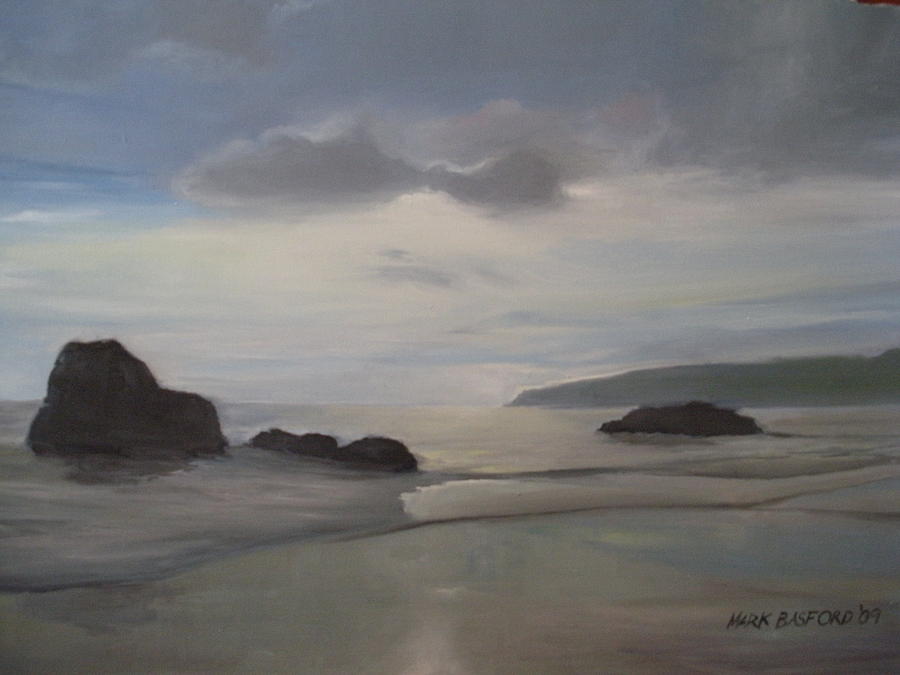This detailed painting by Mark Basford, dated '09, captures a serene coastal beach scene reminiscent of the Pacific Coast. The square, borderless image shows gentle waves washing onto the sandy shore from the viewer's perspective. Large, dark boulder formations punctuate the scene on both the left and right sides, while a few brown rocks peek out of the water. In the distance on the center right, a landmass adds depth to the vista. Above, an overcast sky features an array of big, puffy clouds, some grayish and some aligned with white. Strikingly, moonlight shines faintly from behind one of the clouds, creating a subtle silhouette that intriguingly resembles a shark. The sky's hues transition from a slight blue tint on the top left to a pale pinkish-cream in the center, which beautifully reflects off the water below. This painting, with its artist's signature "Mark Basford 09" on the bottom right, vividly mirrors the tranquil yet dramatic essence of a coastal landscape.